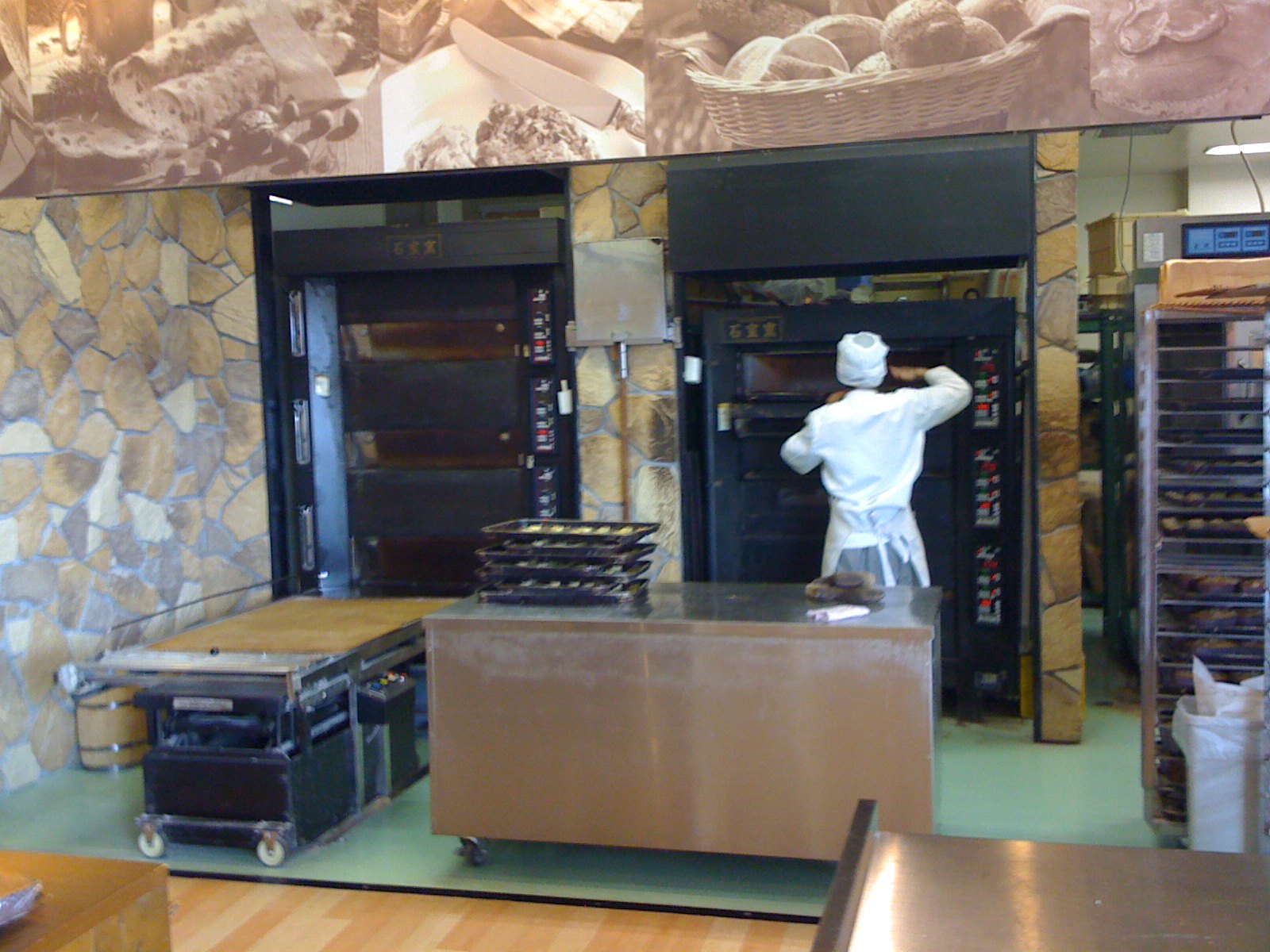The image appears to be set in an industrial kitchen or factory setting. A stone-textured wall can be seen on the left, possibly a wallpaper to mimic stonework. Above the wall runs a large banner or mural depicting various food items such as cheese, bread, and nuts. In the foreground, large industrial ovens, approximately six feet tall, dominate the scene. A man dressed in white kitchen attire and a head covering, though not a traditional chef's hat, tends to one of the ovens, suggesting he might be baking. Several racks, likely holding baked goods, are visible to the right. The green floor contrasts with the sleek, silver metal tables positioned centrally, which hold trays filled with bread or similar baked items. The space exudes a professional and bustling atmosphere typical of a high-capacity kitchen.